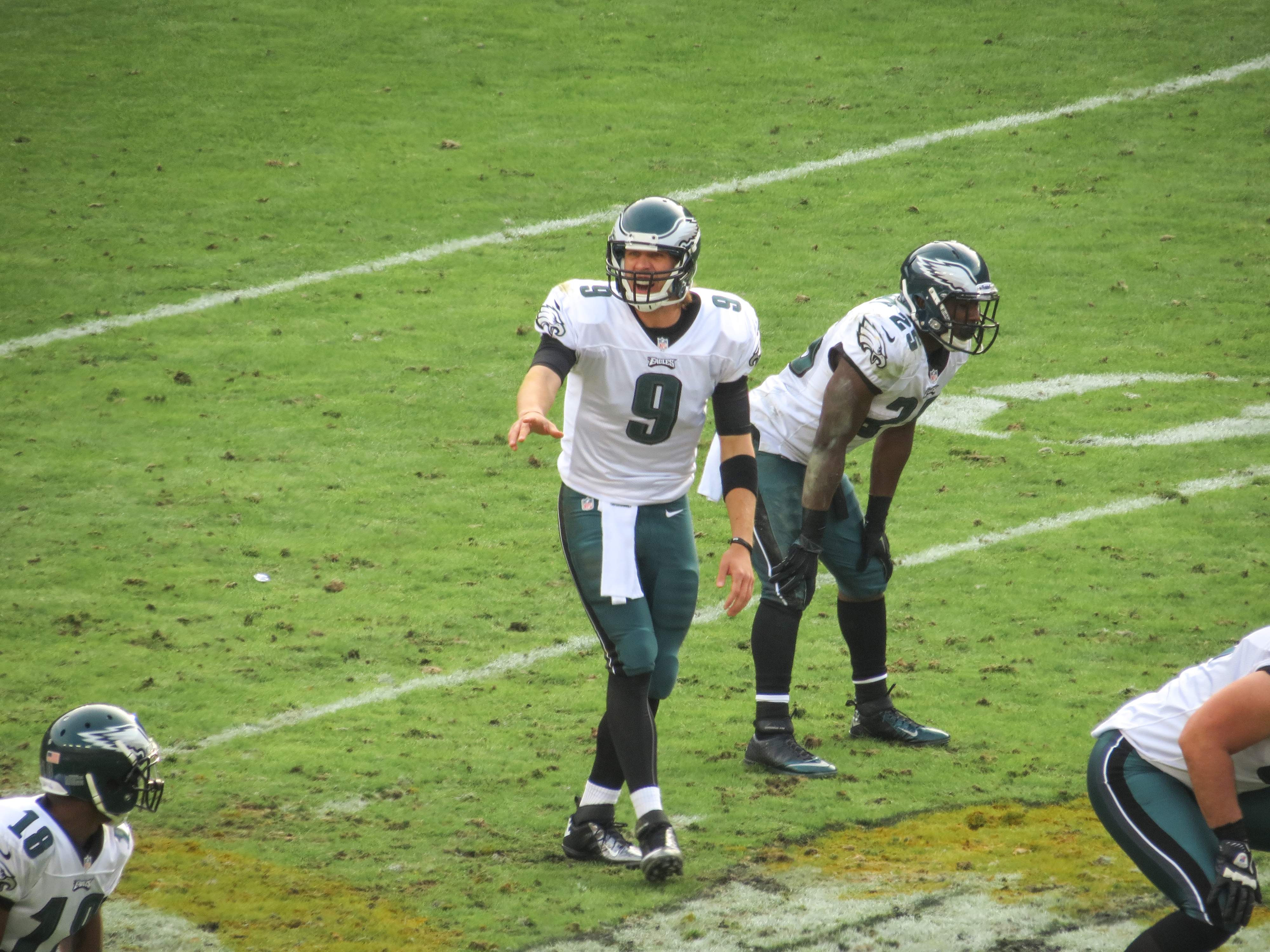The photograph depicts a football game featuring the Philadelphia Eagles, evident from the green and white uniforms and helmets adorned with white wings. The scene showcases four players on a lush green football field marked with white yard lines. Central to the image is the quarterback wearing a white jersey with a green number 9, green pants, black leggings, and white socks. He extends his hand, seemingly shouting instructions, equipped with a black forearm protector and a white towel hanging from his waist. Another player, donned in a jersey with the number 18, appears ready to sprint, while a third stands with his hands on his knees. The background includes visible yard markers, such as the number 0, reinforcing the outdoor setting of the game.